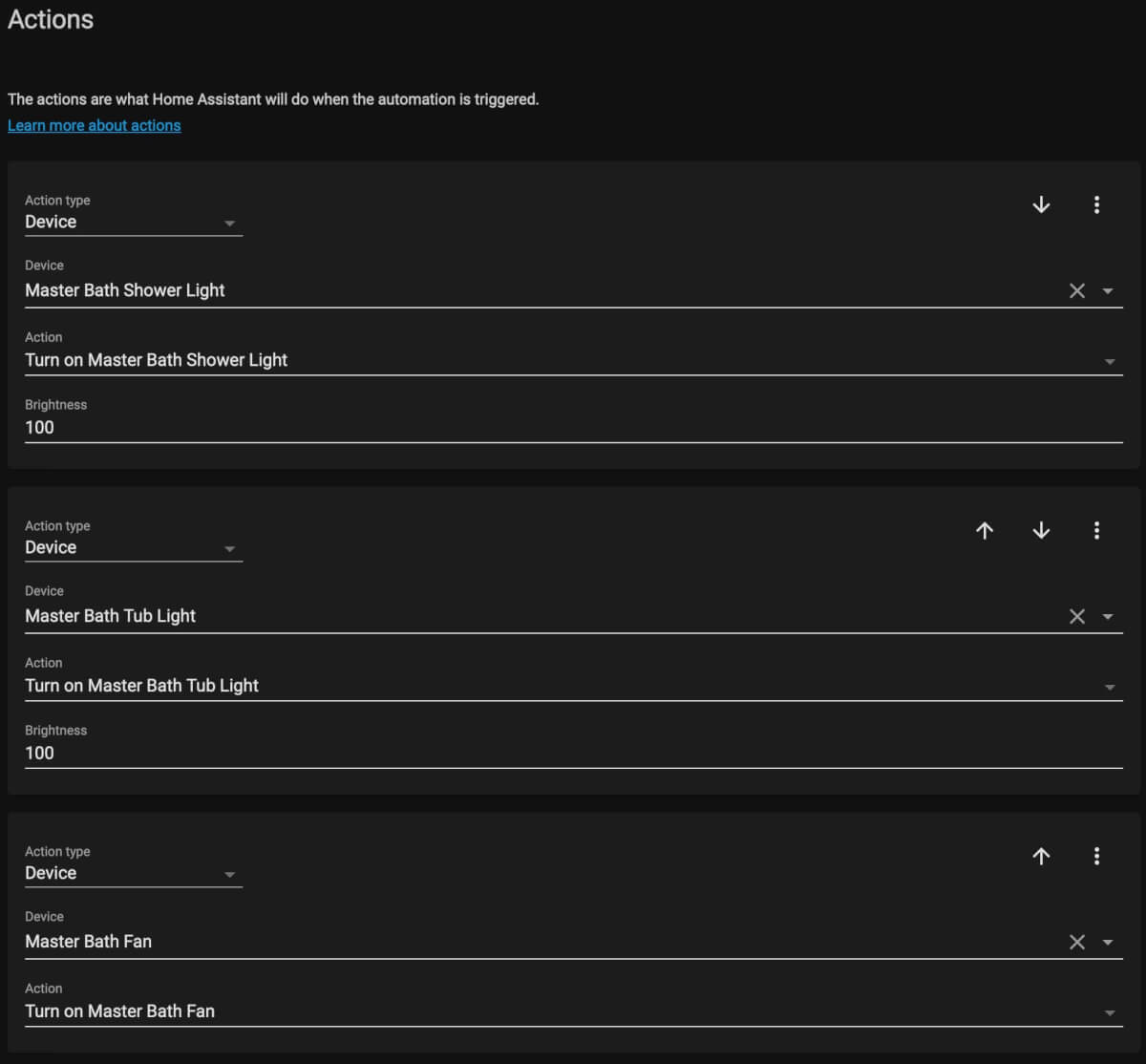This image is a screen capture from the Home Assistant website, prominently displaying a section dedicated to configuring automation actions. At the top of the screen, "Home Assistant" is shown in black, with "Actions" written in white underneath it. The subheading explains that actions define what Home Assistant will execute when a specified automation is triggered.

A blue hyperlink beneath this text reads "Learn more about actions," providing users with additional resources to understand their automation options. Following this, the interface lists various devices and their corresponding actions:

1. **Action Type: Device - Master Bath Shower Light**
   - Action: Turn on Master Bath Shower Light
   - Brightness: 100%

2. **Action Type: Device - Master Bath Tub Light**
   - Action: Turn on Master Bath Tub Light
   - Brightness: 100%

3. **Action Type: Device - Master Bath Fan**
   - Action: Turn on Master Bath Fan

This capture illustrates a comprehensive digital system designed to manage and automate various appliances within a home—specifically focusing on the devices in the user’s master bathroom. The interface allows users to control these devices remotely, possibly via a smartphone, enhancing convenience and efficiency in managing household appliances.